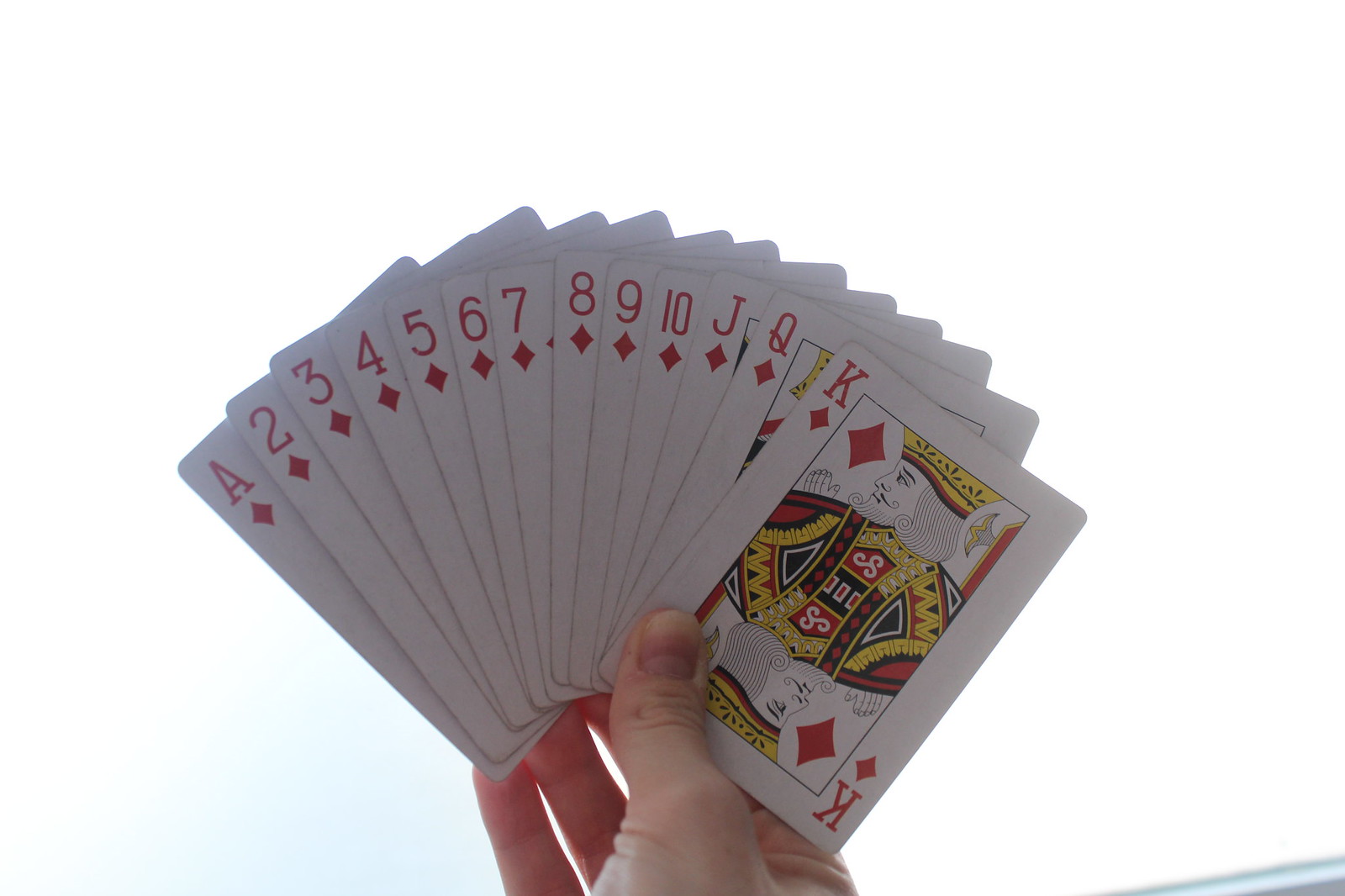In the photograph, a man's right hand expertly holds a perfectly fanned set of diamond cards from a standard deck. The cards, all red and arranged in ascending order from Ace through to King, display an impressive level of precision. The uniformity and the neat spread of the cards suggest that the individual has dedicated considerable time to mastering this skill. The firm grip is indicated by the man’s thumb, whose white-tipped nail stresses the tight hold necessary to maintain the arrangement. The image captures both the dexterity and control required to hold all thirteen cards single-handedly, presenting a remarkable display of card-handling proficiency.